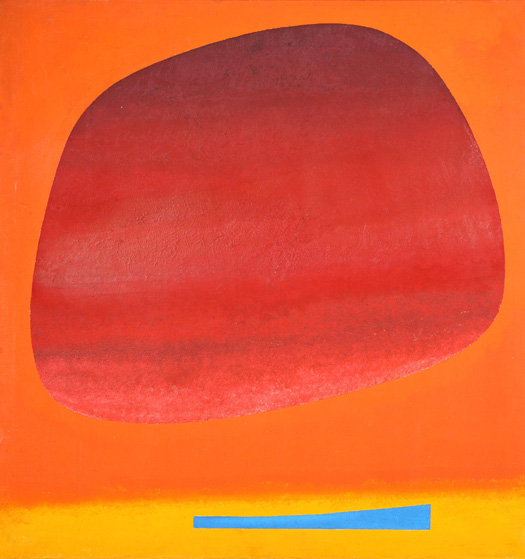The image showcases a modern, contemporary painting dominated by vibrant colors and simplistic geometric shapes. The background is predominantly a gradient of orange, darker at the top and becoming lighter downwards, occupying roughly three-quarters of the canvas. At the bottom, there is a distinct yellow strip, which serves as a base. Central to the composition is a large, red, rhombus-like shape with rounded edges that fills much of the top two-thirds of the image. The red shape features varying shades, from almost black at the top, transitioning through dark red and pinkish tones to whitish red at the middle and bottom, with visible striations adding texture. Suspended on the yellow strip at the bottom of the canvas is a light blue, elongated object resembling a rectangle that expands in width towards the right end. This blue shape is clean, with defined lines, and adds a striking contrast to the warm hues of the background and red form. The painting is devoid of any text, focusing entirely on the interplay of colors and abstract forms.